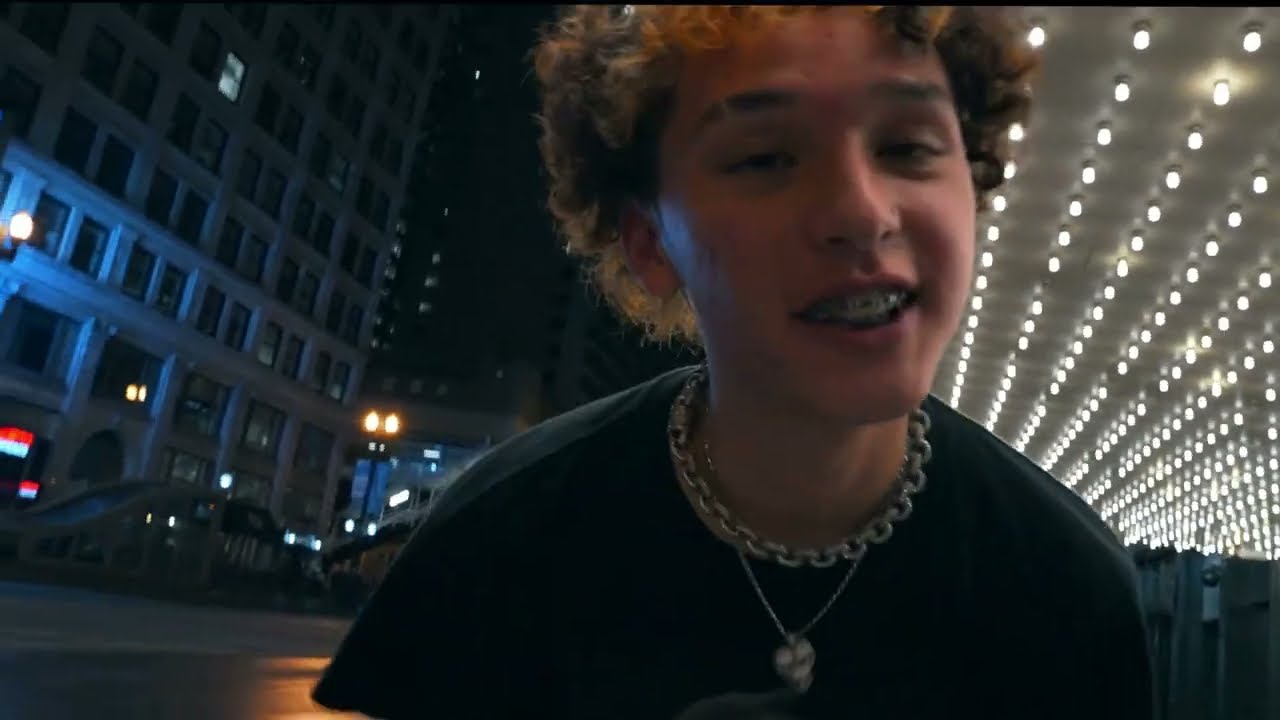The image captures a close-up of a young person with medium-length curly hair featuring black and blondish-orange highlights, whose gender appears androgynous. They have white skin and are dressed in a black t-shirt. Around their neck, they wear a choker-style necklace with a thick chain, complemented by a thinner chain necklace with a pendant. Their facial expression shows them smiling with their eyes partially closed, revealing braces. One eyebrow is distinctively shaved with a lion design. They are leaning forward towards the camera, which is about two feet away, likely standing on a city street at night. Behind their left shoulder is a large pavilion or awning lined with a series of white lights, reminiscent of a theater entrance. The background also features a street with tall buildings, including detailed stone high-rises with numerous small windows, one of which is faintly lit. The setting is dimly lit overall, with globe streetlights visible and possibly a taxi lurking in the shadows.